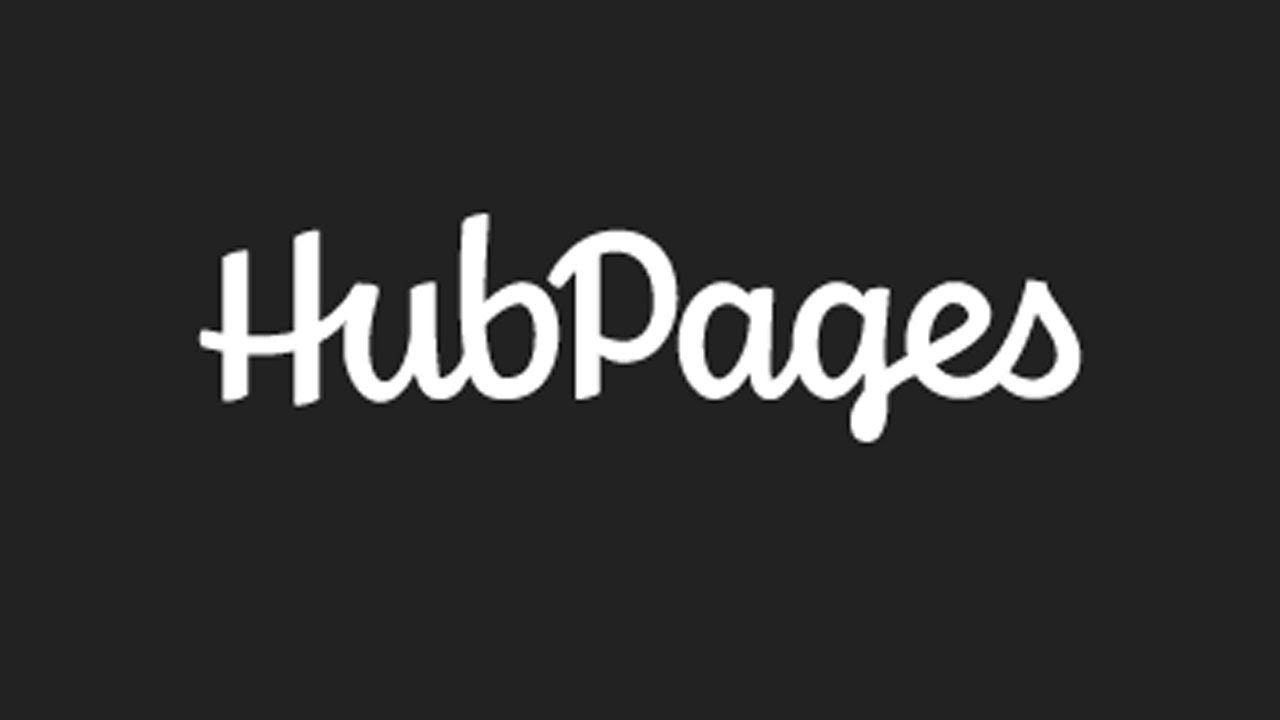The image features a web page banner with a sleek black background. At the center of this banner, the word "HubPages" is prominently displayed in a cursive-like font. This text is written in white and occupies approximately one-third of the banner's height, making it quite large and eye-catching. The word is styled as a single entity with the 'H' and 'P' capitalized, while the remaining letters are in lowercase. The font conveys a casual handwritten appearance, adding a personal touch without being overly ornate. The simplicity of the design—just the black backdrop and the central white text—creates a clean and focused look.